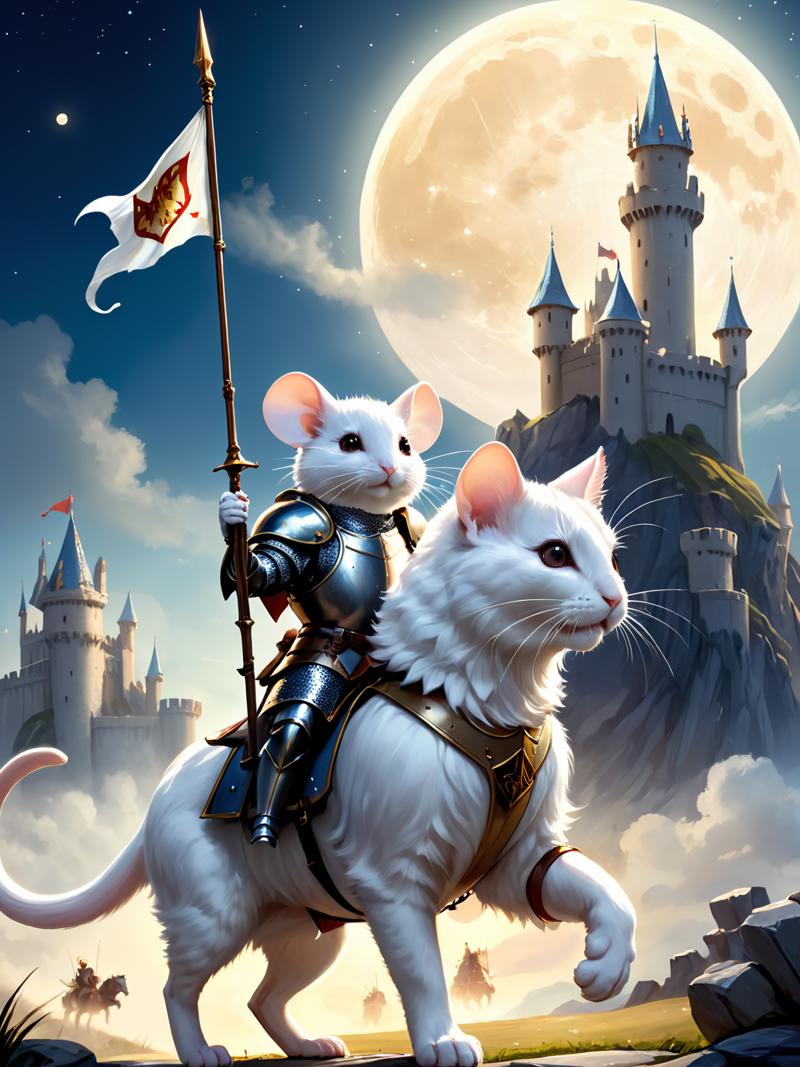This highly stylized, animated digital image features a whimsical, fantasy scenario with detailed elements. The central focus is a white cat wearing a gold brass harness and a saddle, upon which sits a white mouse dressed in human-like knight’s armor. This armor-clad mouse, facing right, wields a spear adorned with a white flag displaying a red symbol of a coat of arms. The cat strikes a heroic pose with its left paw raised.

In the background, a large, luminous full moon illuminates the scene, highlighting a tall castle with blue rooftops and a red flag atop a spire to the left. To the right, another castle appears, intricately built into and atop a mountain. The night sky is filled with stars, clouds, and a bit of fog near the bottom, which partially obscures other knights. These knights, riding horses, seem to be preparing for or riding into battle through a rocky, dusty landscape. The image conveys a rich, fantastical nighttime adventure with knights, castles, and mystical creatures under a brilliant moonlit sky.